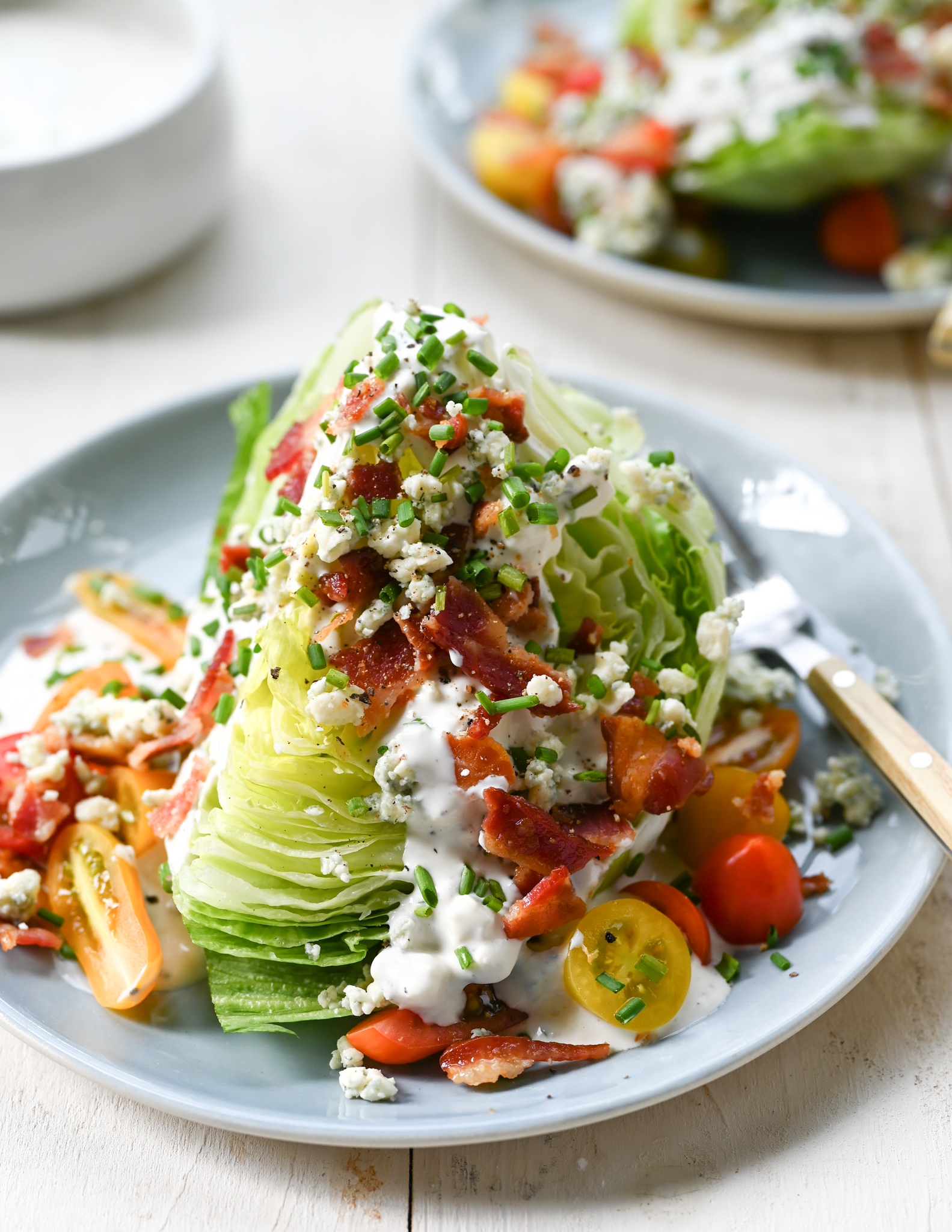This professionally photographed image showcases a meticulously prepared Cobb salad presented on a light grayish-blue plate with a silver-handled fork resting on its right. The salad features a vibrant array of ingredients, including a chunk of lettuce placed upside down on the plate, halved cherry tomatoes in both red and yellow, crumbled blue cheese, and crispy bacon bits with a rich dark red hue. The salad is drizzled with either ranch or blue cheese dressing and garnished with finely chopped chives or parsley. This colorful presentation sits on a table made of wide wooden boards painted white, adding a rustic charm to the scene. In the background, a slightly blurred second salad plate and a white bowl, possibly containing extra dressing, further enhance the image's depth and focus on the main dish. The composition's color palette and arrangement emphasize the culinary artistry, making the salad the striking focal point.